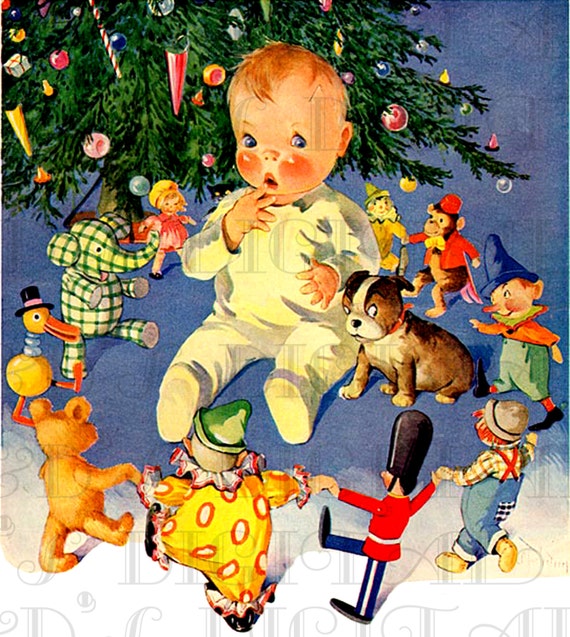The vintage artwork depicts an adorable scene of a baby surrounded by various animated toys dancing in a circle. The baby, wearing an off-white onesie that covers its feet, has red hair, blue eyes, and rosy cheeks, and sits with a finger to its mouth, displaying a confused expression. Next to the baby, on its left, is an exceedingly small puppy with a red collar. The puppy, primarily brown with a distinctive white stripe through the center of its head, around its muzzle, and on its belly, sits on its hind legs, looking bewilderedly at the dancing toys. These playful toys, including bears, ducks, toy soldiers, clowns, and monkeys, create a lively atmosphere. Behind the baby and toys stands a decorated Christmas tree with a red stand, contributing to the festive setting of the image. The Christmas tree is lush and green, adorned modestly with winter-themed decorations. There is a faint, unreadable watermark in the background, adding to the vintage charm of the piece.